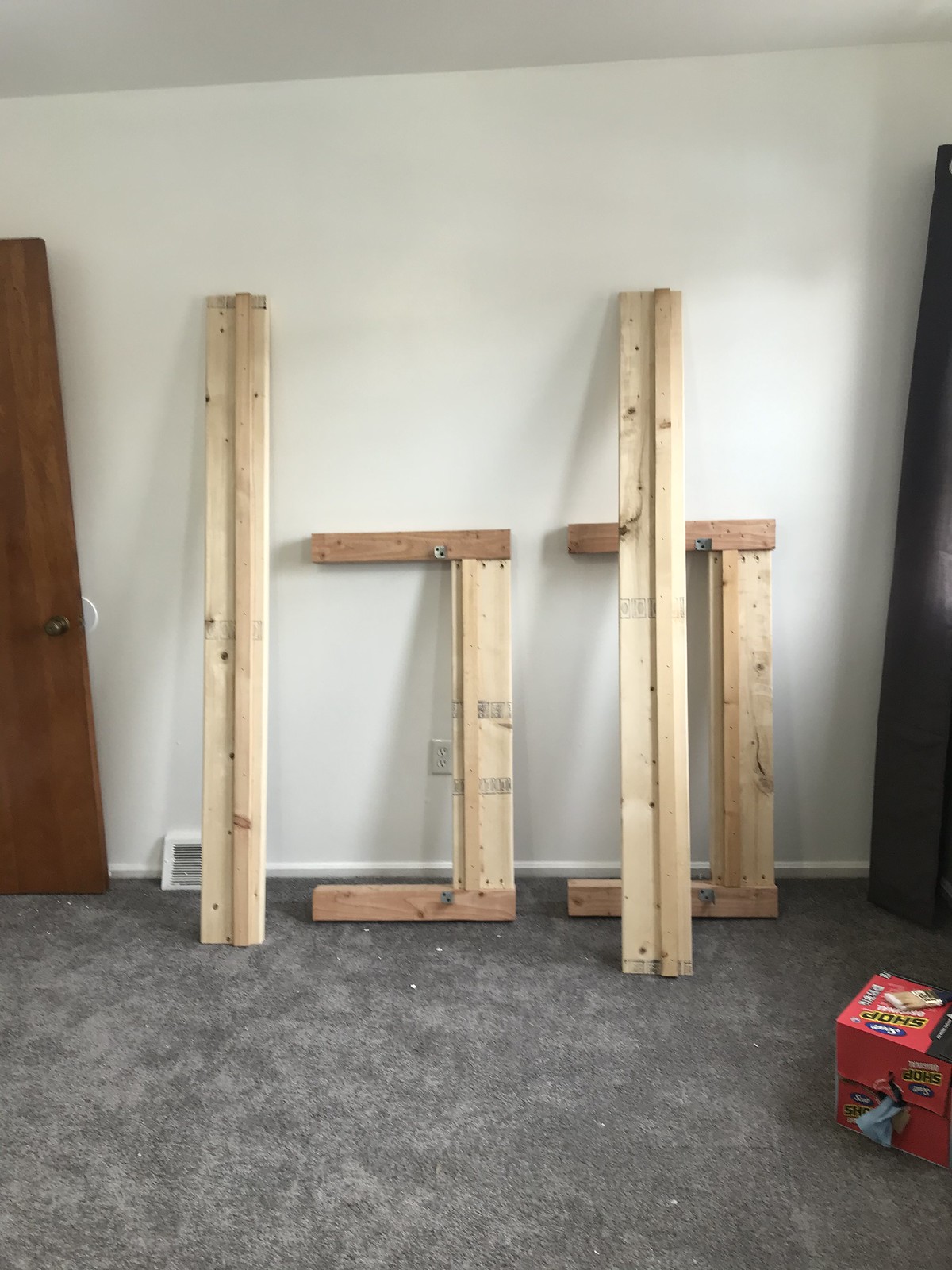The image depicts a room that appears to be undergoing renovations or the assembly of furniture, possibly a bed frame. The room is roughly twice as high as it is wide, featuring a floor covered in gray carpeting that varies in shade from medium to light gray, depending on lighting and carpet positioning. An off-white wall serves as the backdrop, with a medium-stained wooden door to the left, which is open. 

Propped against the wall are several pieces of light-colored wood, likely components of a disassembled bed frame. These include four two-by-fours, nearly reaching the height of the door. Between these wooden pieces are two structures resembling backwards "C" shapes, one positioned slightly to the left and the other behind the two-by-fours on the right.

In the bottom right corner of the image, there is a red cardboard box labeled "shop rags," with a paintbrush possibly resting on top. An electrical outlet is visible in the middle of the wall, and the gray carpet is somewhat messy, with some wood pieces and possibly other debris scattered about. This scene suggests an ongoing setup or moving-in process.